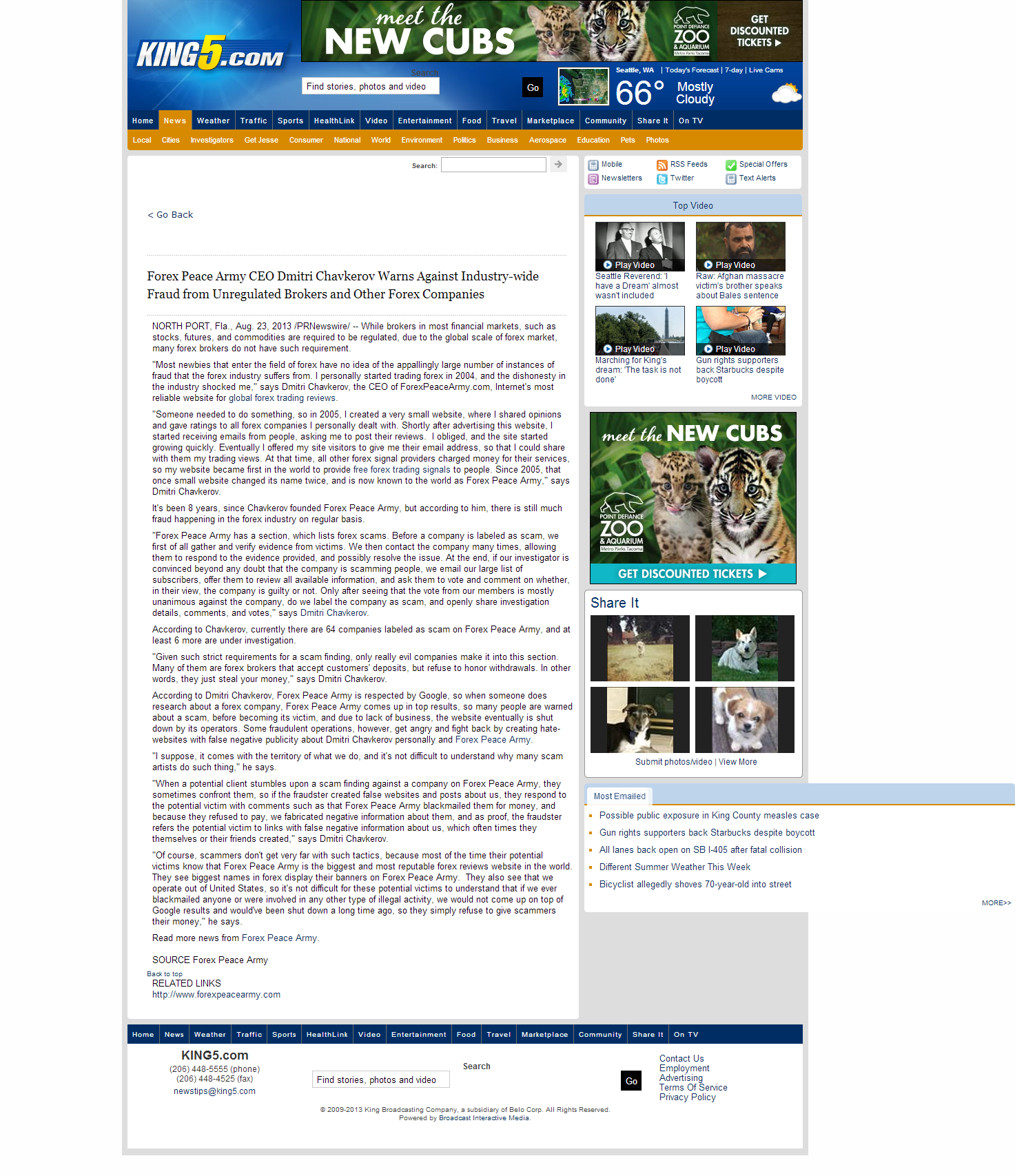This is a vertically-oriented rectangular image featuring various design elements and text.

At the top center, lowercase script in white font reads "meet the." Directly below, in bold white capital letters, it says "NEW CUBS." Flanking this text are images of two young big cats, emphasizing that they are cubs. Adjacent to this, there is a small logo of an animal, outlined in white, accompanied by the text "ZOO" in all capital letters, white font. Next to the logo, there's a small brown area with bold white capital letters stating, "GET DISCOUNTED TICKETS."

The left side of the page features a blue background that extends underneath the "new cubs" section, creating a seamless transition. On this blue background, text in all capital white letters reads "KING," followed by the number "5" in yellow, and then "COM" in white once more.

In the main content area, there are navigational menu options displayed across the top on a darker blue background with white font. The second option in the menu is highlighted in a yellow-orange color, indicating it is selected. Beneath this darker blue bar are additional menu options in the same yellow-orange color. 

On the white background covering the main area, an article section begins on the left side. The headline reads "FOX [incomplete text]," followed by "Peace Army CEO," and a name, warning against industry-wide fraud from unregulated brokers and other companies. The article text itself is too small to be legible. To the right of the article are some images that complement the content.

A blue bar at the bottom of the page contains more menu items, providing further navigation options.